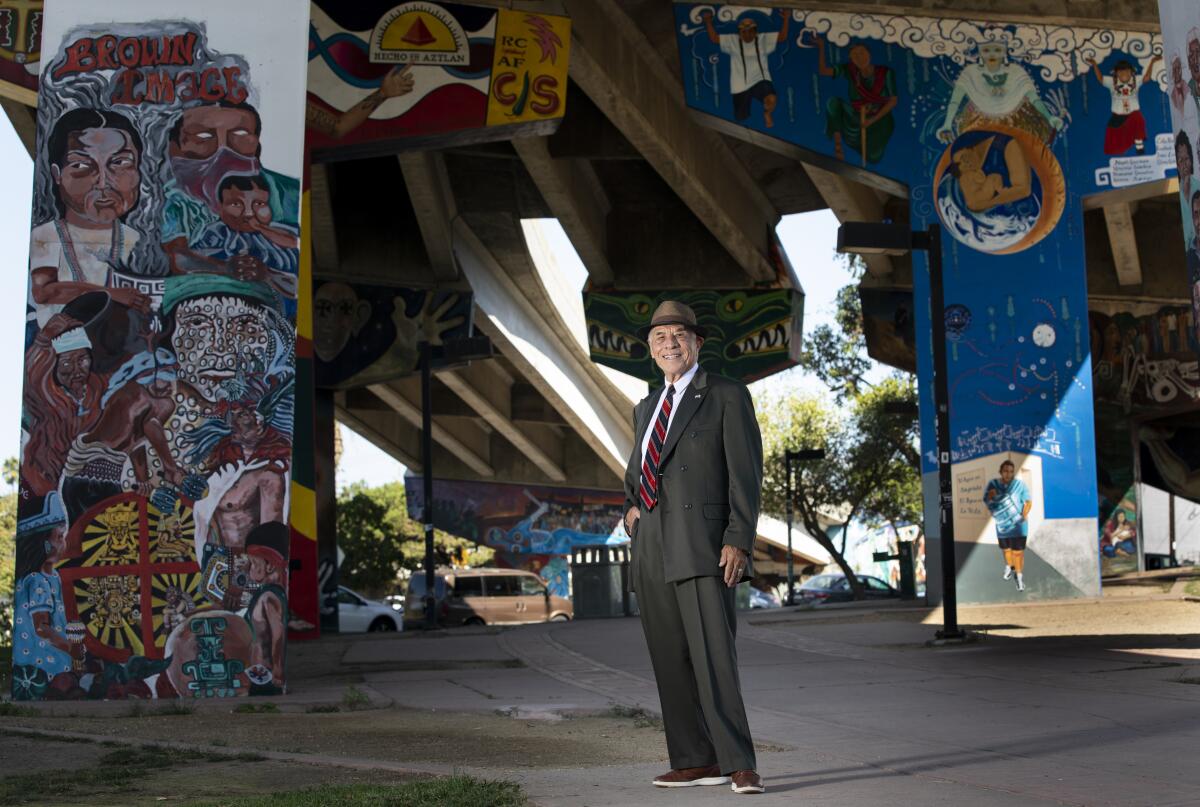In this vibrant and detailed photograph, an older man stands confidently under an overpass adorned with colorful murals. He is wearing a distinctive brown fedora hat, a black suit jacket, and gray pants complemented by a red and black striped tie over a white shirt. His brown shoes complete his stylish ensemble. The man's left hand displays a piece of jewelry, while his right hand is casually tucked into his pocket. 

The overpass's concrete structure is decorated with various expressive murals. On the left pillar, a mural features multiple characters' faces, with the phrase "brown image" prominently displayed. To the right, another pillar showcases a blue background with four figures at the top and one at the bottom, with white stars scattered across. Nearby, another mural includes green animal figures, possibly alligators or lions, with stark white teeth. Yet another column features figures that seem to be lifting the sky, set against a blue sky with white clouds and raindrops. Other highlighted motifs include a red triangle on a yellow background and a DNA-like symbol with blue and reddish-blue colors.

The ground beneath the man is gray cement, edged with brown dirt and patches of green grass. Beyond the overpass, the area includes several parked cars, hinting at a busy urban setting with green trees providing a backdrop. The detailed graffiti and murals, combined with the man’s poised presence, suggest this underpass is a frequented and lively spot despite being beneath a bridge.